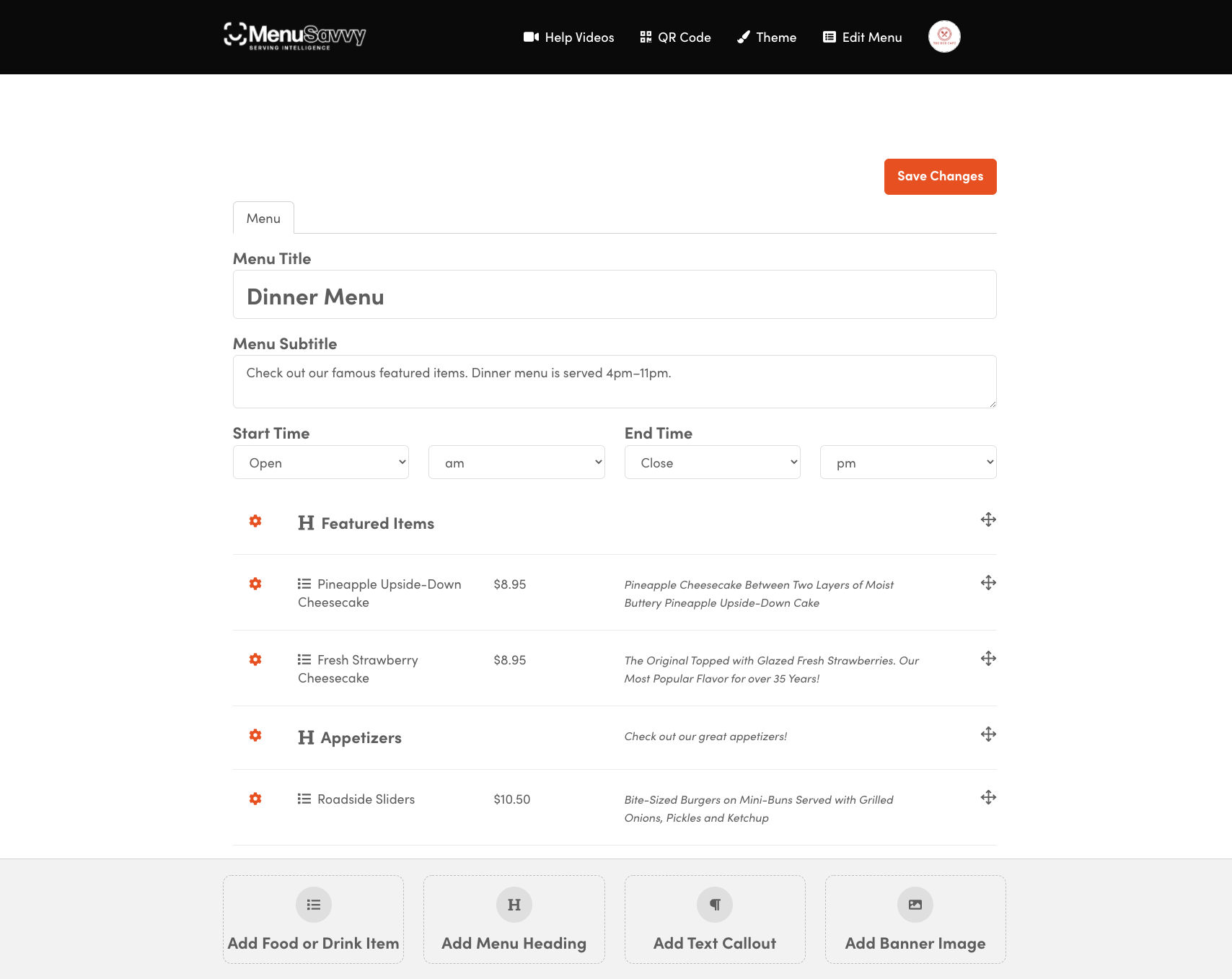In the image, the top section prominently displays "Menu Savvy" along with helpful options such as "Help Videos," "QR Code," "Theme," and "Edit Menu." There is an orange button labeled "Save Changes" beneath these options. The menu section is titled "Dinner Menu" with a subtitle that reads "Check Out Our Famous Featured Items." The operation hours for the dinner menu are listed as serving from 4 PM to 11 PM. Despite the blurriness, additional text includes fields labeled "Start Time" and "End Time," designated as "Open AM" and "Close AM" respectively. The featured items section includes delectable offerings such as "Pineapple Upside Down Cheesecake," "Fresh Strawberry Cheesecake," and under appetizers, items like "Roadside Sliders." The image contains another mention of "Pineapple Upside Down Cake" and references the popularity of certain original menu items, although specific details remain unclear due to the blurry quality.